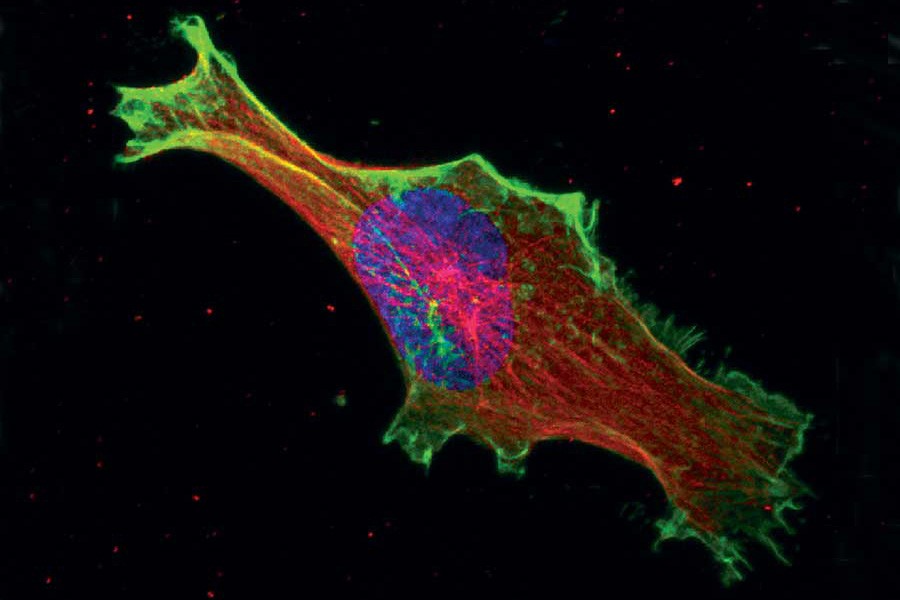This intriguing image resembles a firing neuron or an otherworldly creature, set against a stark black background filled with red and green speckles. At the center, an oddly shaped form stands out, outlined in bright neon green light. The interior of this form features a circle of bluish-purple with red accents, surrounded by strands of red that transition into yellowish-green, blending into the neon green edges. While the shape itself is undefined and could evoke the appearance of a neuron or even a fantastical dinosaur with enormous teeth, the striking contrast and vibrant colors create a mesmerizing, almost cosmic scene. The surrounding red and green speckles contribute to a celestial feel, enhancing the image's mysterious and abstract nature.